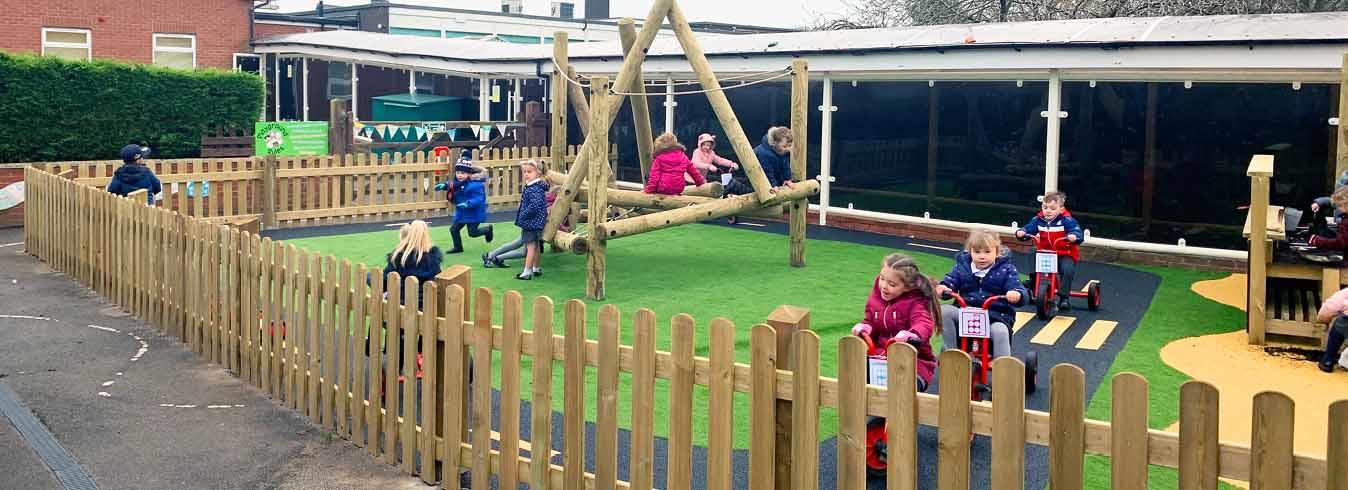This is a detailed photograph of a vibrant children’s outdoor playground, likely at a school, depicted in a longer-than-tall format. About fifteen children, ranging in age from three to five years old, are energetically playing within the gated area outlined by a roughly three-foot-high natural wooden fence. The ground is covered with astroturf, which is notably green and mimics the appearance of grass, potentially featuring a racetrack design. 

On the left side of the playground, children crawl over a structure made of logs, while on the right, three kids ride red tricycles, reminiscent of big wheels, near a wooden structure with a yellow backdrop. In the midst of their activities, some children are seen running around. The season appears to be winter, as reflected by the colorful coats, including a little girl in pink and a boy in blue, worn by the children. 

The backdrop of this lively scene includes a red brick school building equipped with an awning providing shelter from the rain and adjacent pavement outside the fenced area. The setting is naturally bright, indicating a clear day, complemented by visible trees and a portion of the bright sky in the background. The image is clear and full of activity, capturing a joyous recess moment.